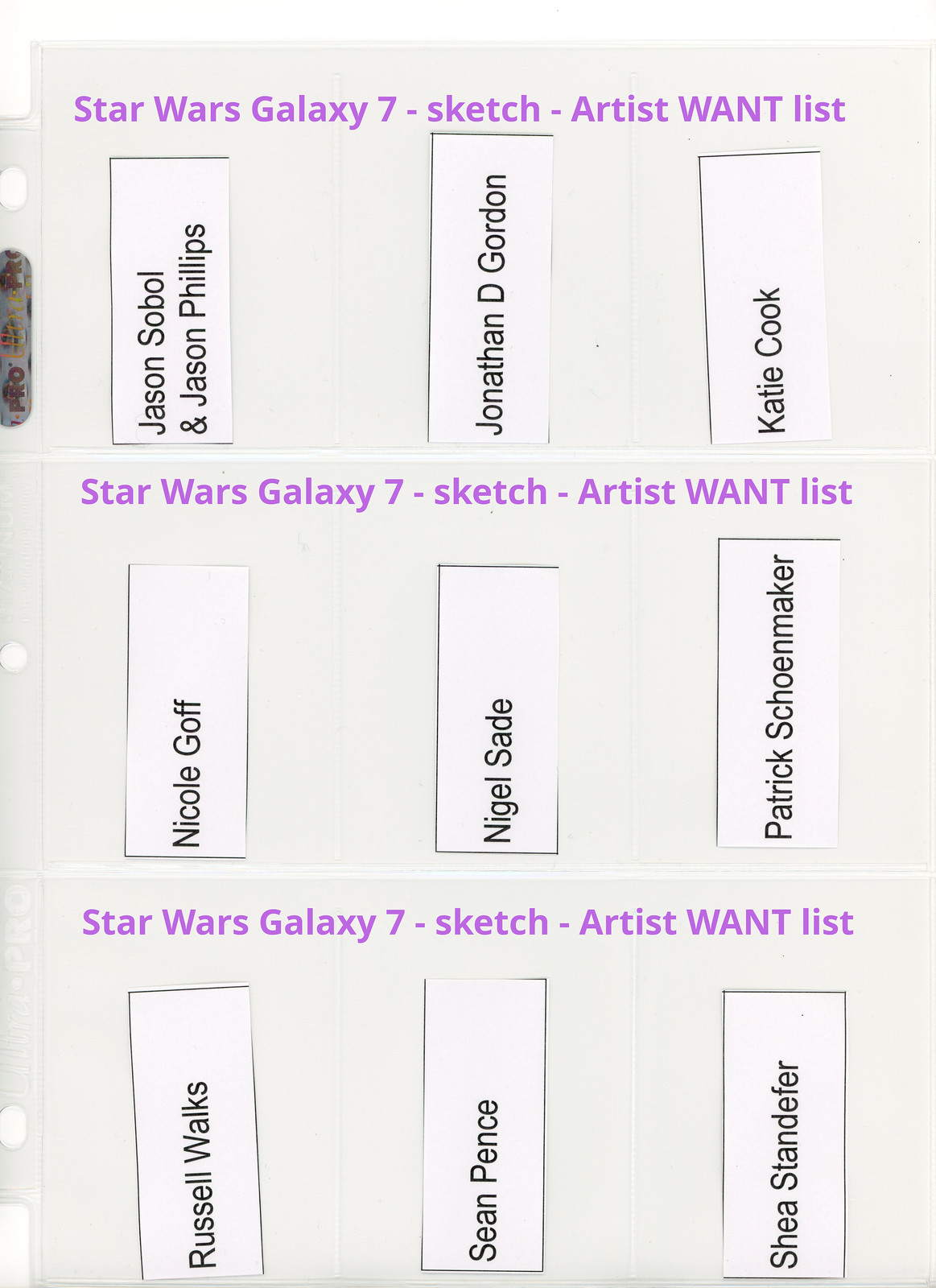The image is an off-white background with the purple heading "Star Wars Galaxy 7 Sketch Artist Want List" repeated three times, once at the top, once in the middle, and once at the bottom. Each section contains a list of names on small slips of white paper with black print. These slips are oriented vertically, requiring the viewer to turn their head 90 degrees to the left to read them properly. There are three rows of these name slips, with three names in each row, totaling nine names. The listed names are in the order of Jason Sobel, Jason Phillips, Jonathan D. Gordon, Katie Cook, Nicole Goff, Nigel Sade, Patrick Shoemaker, Russell Walks, Sean Pence, and Shaya Standifer. Additionally, in the upper left corner of the image, there's a hologram sticker, reminiscent of those used on card protectors.